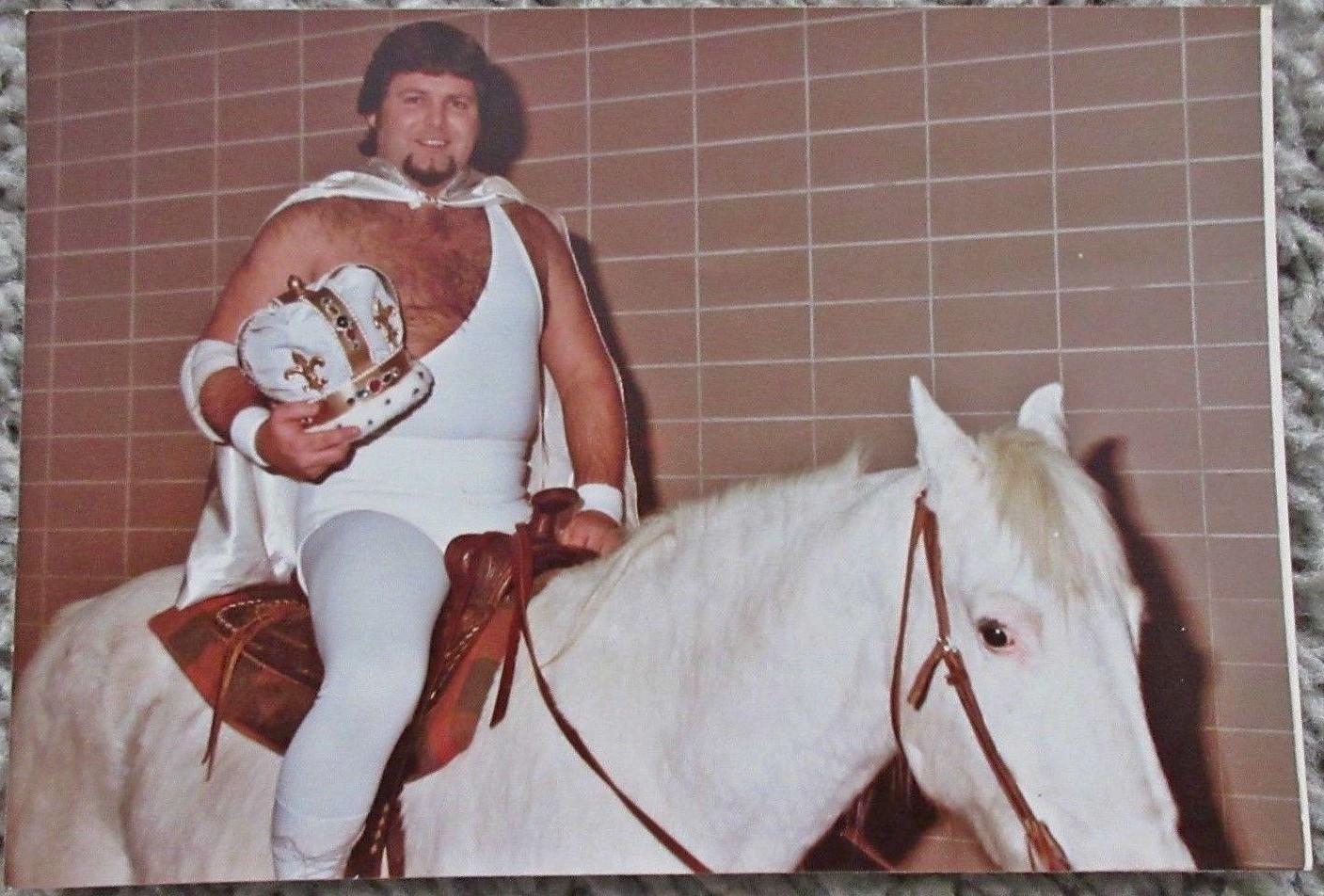In the image, a man, who appears to be a wrestler, is confidently seated on a white horse. The horse, adorned with a saddle and a bridle with reins, is positioned dead center in the middle of the photograph, against a background of a tiled wall. The man, slightly to the left of center, is dressed in a striking Greek or Roman-inspired costume, consisting of a white cape, white tights, and white underwear or short shorts over the tights. His attire also includes a unique tank top with only one sleeve, revealing his very hairy chest.

The man, who has dark brown hair with straight-cut bangs and a goatee, is smiling warmly. He proudly carries a crown, which is white with gold decorations, in his hand. The colors in the image include shades of pinkish brown, beige, gold, black, white, various shades of brown, and hints of red. The horse, appearing calm and obedient, stands quietly under the man’s firm yet gentle grip on the reins. The overall setting of the photograph suggests a sense of grandeur and historical influence, emphasized by the detailed and dramatic costume worn by the man.